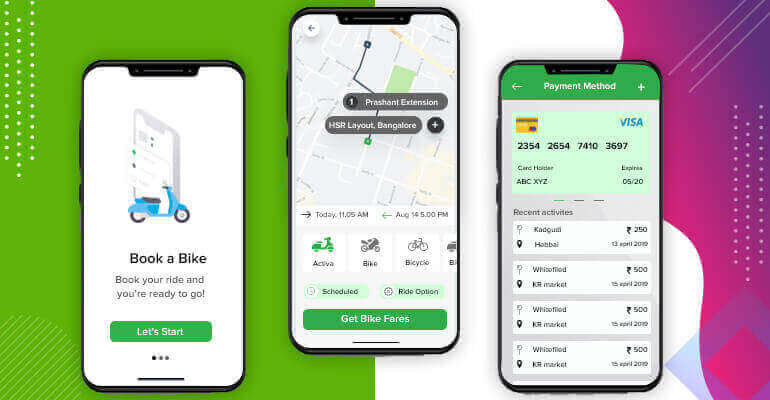The website showcases a mobile app designed for booking motorbikes or bicycles. The homepage prominently features three smartphone images, each depicting a different function of the app.

- **Left Phone Display:** This screen appears to be the app's main entry page, greeting the user with an icon resembling a bike or Vespa, set against the background of a smartphone. Below this icon, the text "Book a Bike" and "Book your ride and you're ready to go" is displayed. There's a "Let’s Start" button beneath the instructions, accompanied by three dots suggesting that users can scroll through a carousel of images or features.

- **Center Phone Display:** The focus here is on a map showing two marked locations, illustrating the function to choose pickup and drop-off points. Additional options appear for selecting the time and type of bike, such as "Active," "Bike," or "Bicycle." Beneath these choice selectors are buttons labeled "Schedule Ride" and "Get Bike Fares."

- **Right Phone Display:** This screen provides a view of the payment methods, including an image of a credit card. Below this, there are four boxes under the "Recent Activities" heading, listing the start and end locations, fare amounts in rupees, and corresponding dates for previous rides.

This detailed representation effectively conveys how the app functions from initial booking to payment, guiding users through each essential step.